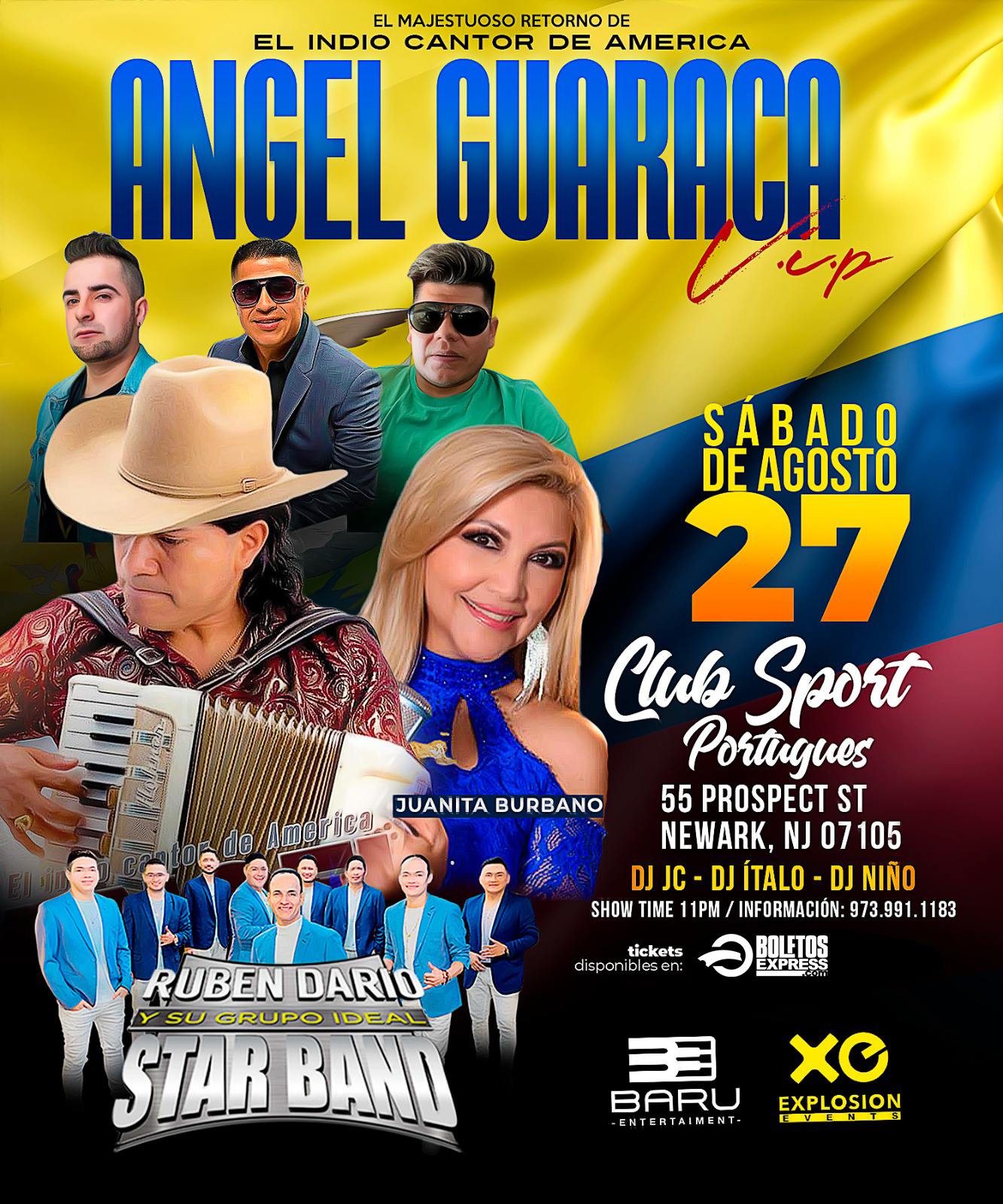This vibrant event poster advertises a concert for "Angel Guaraca VIP," taking place on Saturday, August 27, at Club Sport Portuguese, 55 Prospect Street, Newark, New Jersey, 07105. The background of the poster features a bold tricolor design with yellow, blue, and red stripes. The headline text is blue and prominently features the names "Angel Guaraca" alongside titles such as "Miguel Magistroso" and "Retono de El Indio, Cantor de America."

The upper section of the image showcases a group of performers. In the back row, three men stand, while in the front, a man wearing a cowboy hat plays an accordion. Beside him, a smiling blonde woman in a blue dress with long silver earrings adds a touch of elegance to the scene. At the bottom of the poster, approximately nine additional band members are shown, adding to the festive and musical atmosphere. The text below identifies the ensemble as "Ruben Dario Y Su Grupo Ideal Star Band."

Additional details include the start time of the event, 11 p.m., and a contact number for more information: 9739911183. Logos of various sponsors appear at the bottom right of the poster, indicating a broad support network for this likely lively and culturally rich celebration.